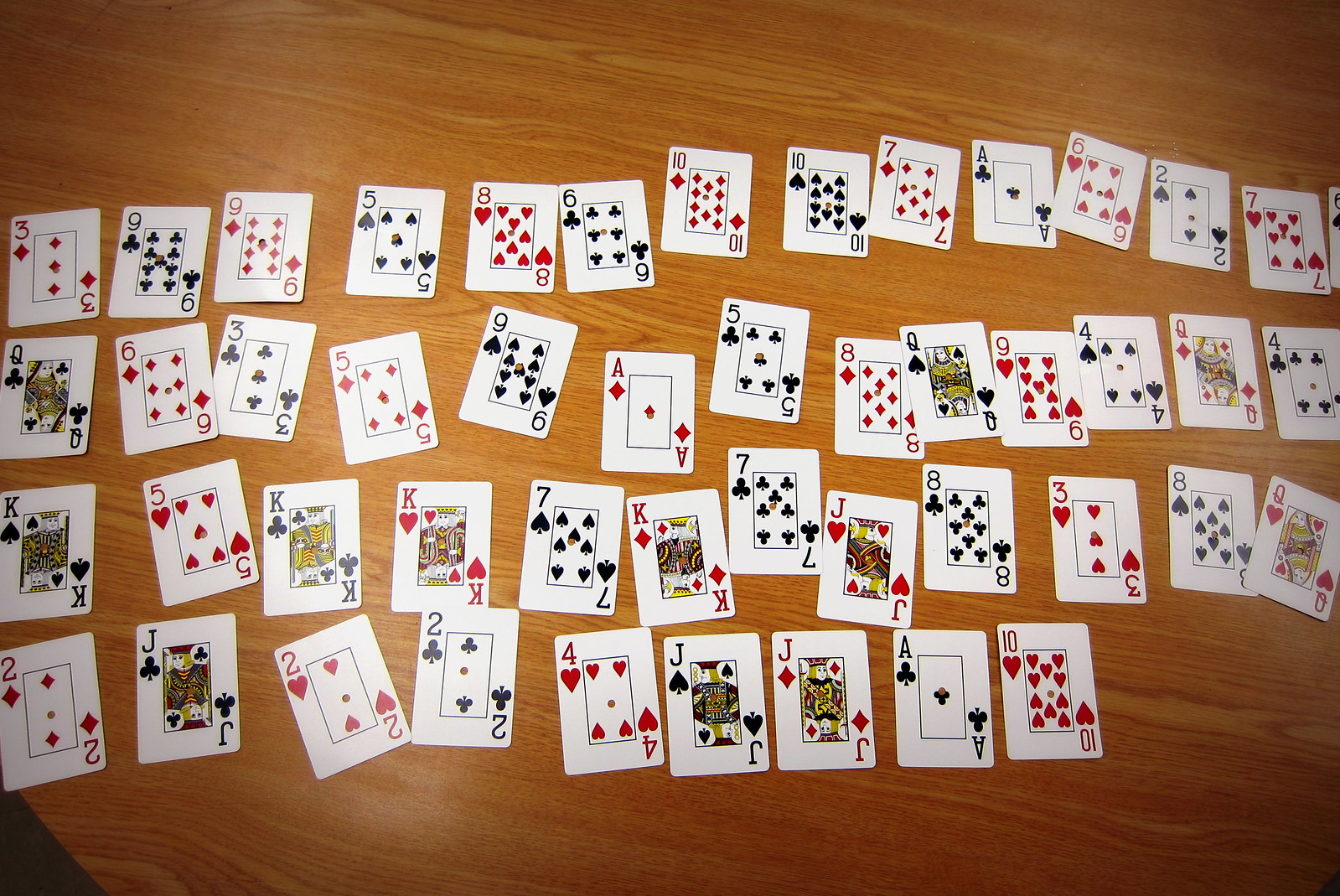A warm, cherry wood tabletop with prominent horizontal grain lines provides the backdrop for an intricately arranged array of playing cards. The cards are organized into four roughly aligned rows. The first three rows each contain approximately 12 to 13 cards, while the fourth row holds only nine. Each card is turned face up, displaying a variety of suits including diamonds, spades, hearts, and clubs. Amidst the mix, a few jokers, kings, and queens are also prominently visible, adding a touch of regality and intrigue to the setup. The overall scene gives the impression of a meticulously planned card game or a whimsical display of collectible cards.